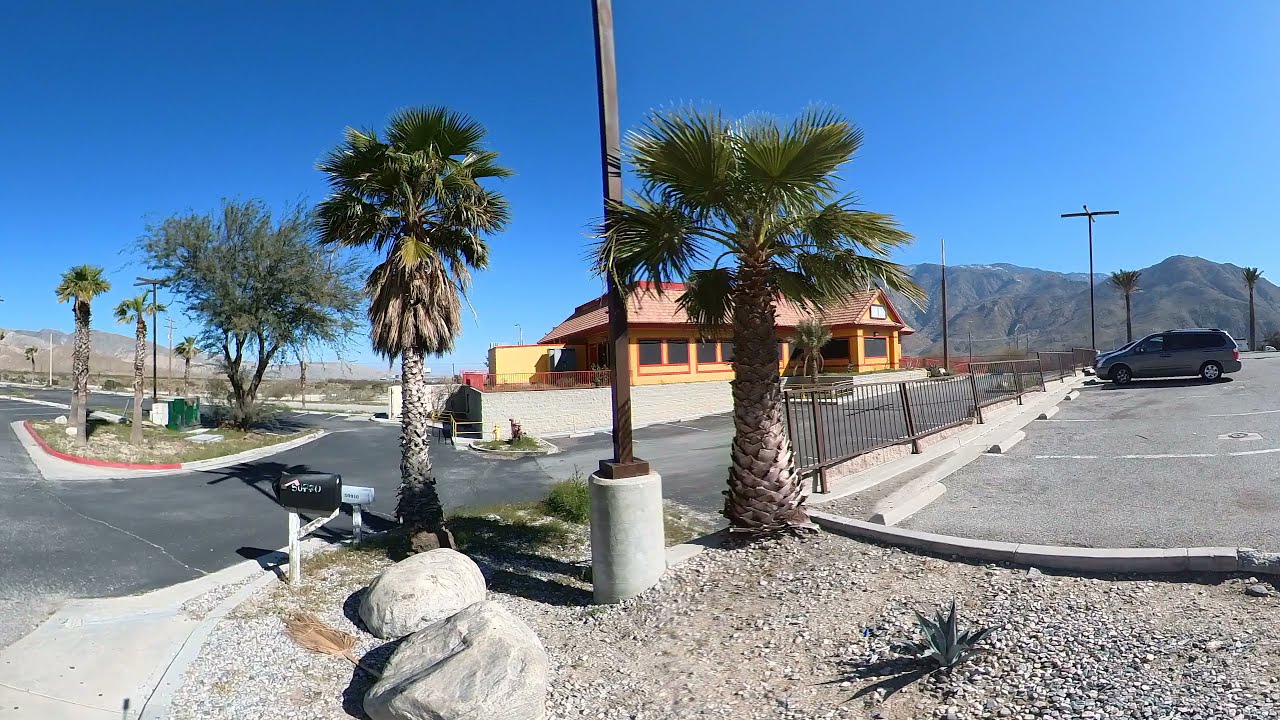In this image, a vibrant urban scene is depicted against a backdrop of a clear, blue sky and distant mountain ranges. At the center, a rectangular garden section features a pair of tall palm trees flanking a significant concrete pole, whose top is out of view. The garden, set within a city landscape, comprises a combination of gray rocks and assorted greenery, including trees with white or green-yellow leaves. Surrounding this centerpiece is a parking area marked with white and red curbs and lined with several vehicles, including a gray van.

Prominent in the background is a single-story building with an orange-red roof and yellow-red exterior walls. This structure, possibly a restaurant with a drive-thru, presents dark windows and a guarded perimeter. Adjacent to it are two distinctive mailboxes, one black and one white, along with a green junction box.

The entire setting is accentuated by hills with patches of green grass and grayish-brown hues, enhancing the urban tableau with a touch of natural beauty on a bright, sunny day.